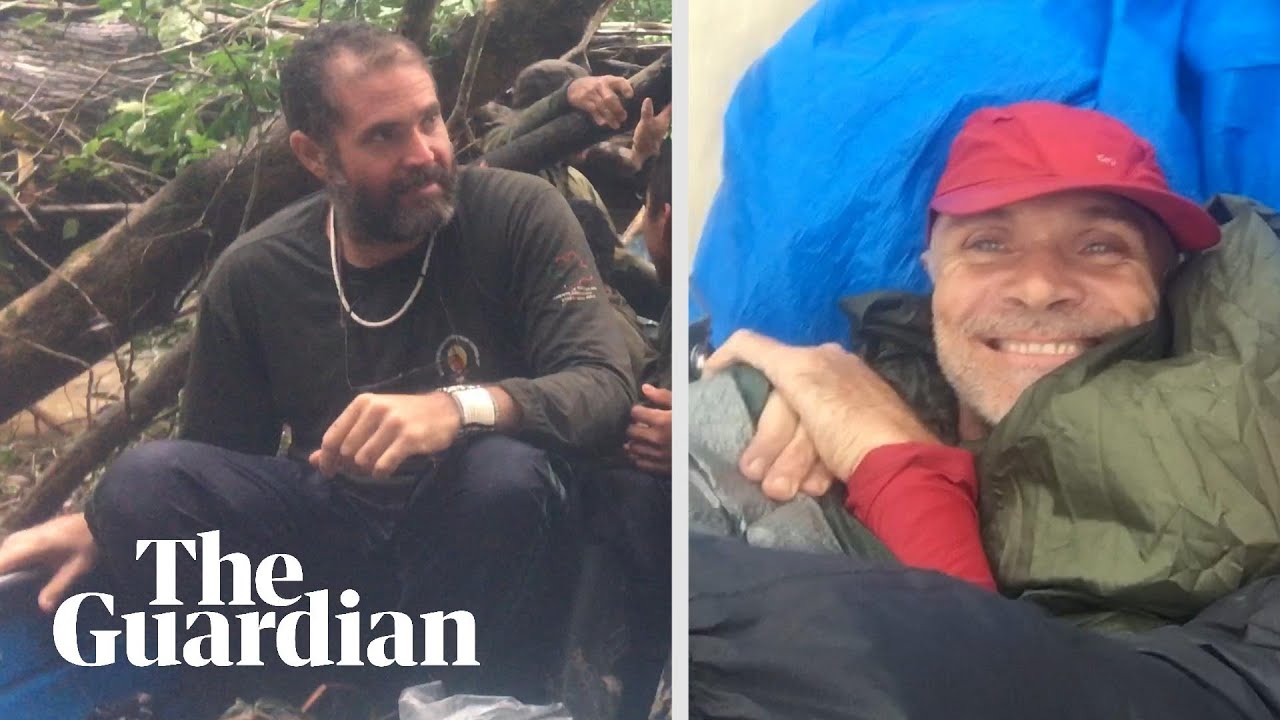The image from "The Guardian" is divided into two sections, juxtaposing the same middle-aged Caucasian man at different points in his life. On the left, he is depicted in a forest setting, squatting or sitting among trees, leaves, and partially obscured figures of other people. He sports a full beard, short hair receding from the front, and is attired in a long-sleeved green shirt paired with navy or dark pants and sneakers. He accessorizes with a large silver or gold necklace and a watch, and clutches something blue in one hand. His posture is relaxed, and he gazes into the distance.

Conversely, the right section portrays a more aged and frail version of the same man, possibly indicating a dramatic shift in circumstances, perhaps homelessness. He lies on a blue tarp or similar material, partially covered by a green jacket, blanket, or sleeping bag. He wears a red baseball cap and a matching long-sleeved shirt, smiling despite his evidently diminished and slimmer appearance. The comparison between the two images illustrates a stark contrast, suggesting a narrative of decline or hardship.